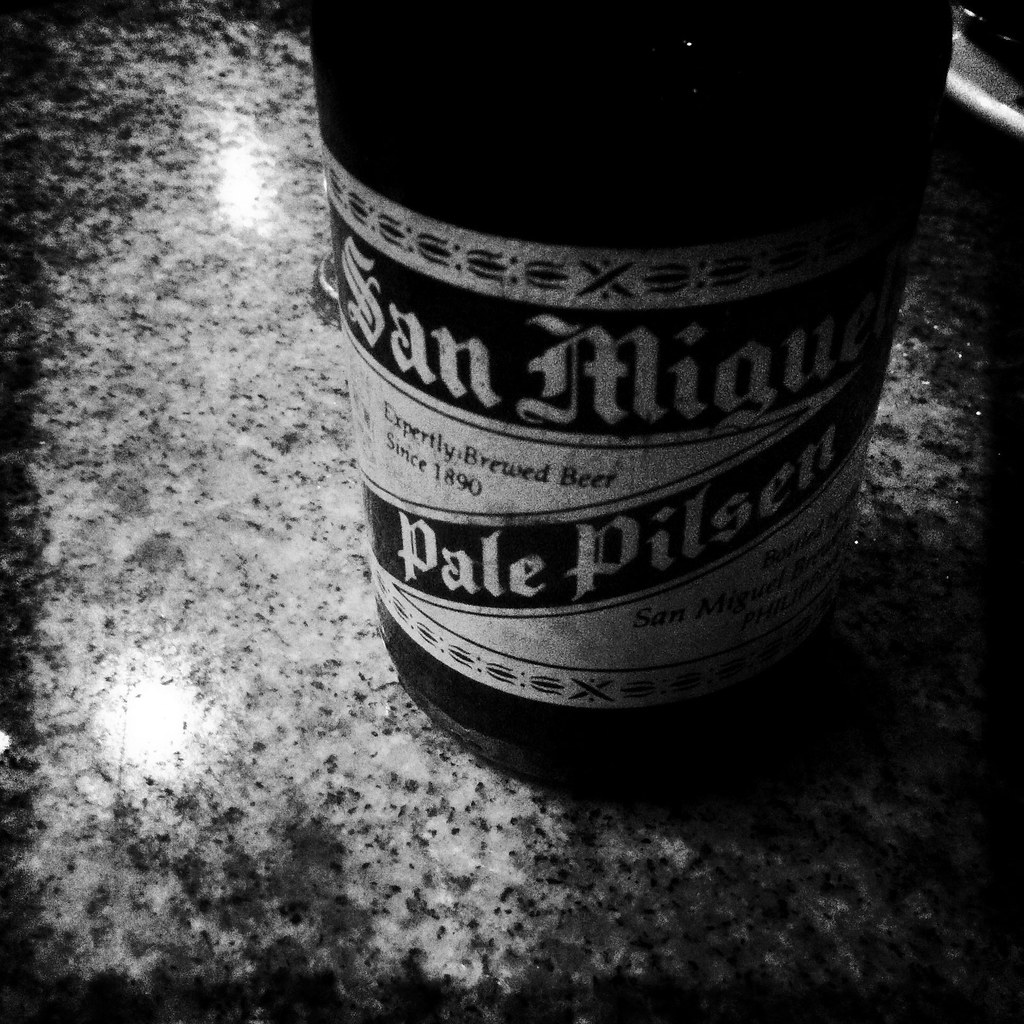This is a square-format black and white photograph featuring the midsection of a dark-colored beer bottle prominently occupying about two-thirds of the image height, positioned on a shiny, gray speckled or granite countertop. The bottle is partially visible, cut off near the neck. The white label on the bottle, horizontally oriented, is detailed with several forms of typography. At the top of the label, a decorative border is visible above a black horizontal band featuring the white Gothic text "San Miguel." Below this, on the white portion of the label, the black text reads "expertly brewed beer since 1890." Further down, a rectangular black band, tilted from the bottom left to the top right of the label, displays the words "Pale Pilsen" in white Gothic script. Additional illegible text is present at the lower section of the label, with another decorative border at the bottom. The simple and focused composition highlights the iconic branding and design elements of the beer bottle.